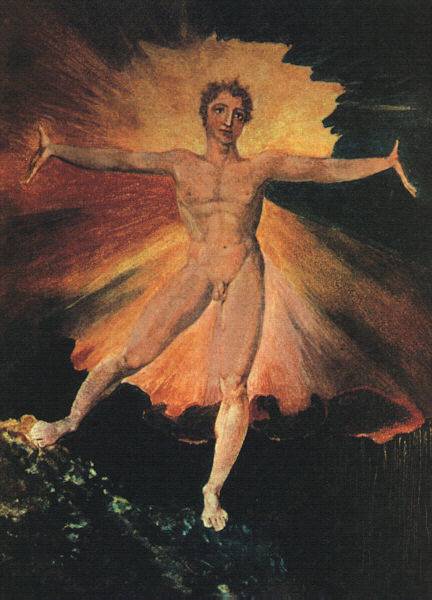This image is a detailed and abstract painting of a nude man standing with his legs spread. His left leg is straight beneath him, while his right foot rests upon a small, elevated brown stone on a green surface. The man stands with his arms fully extended to the sides, reminiscent of a crucifix pose. He has short hair, and although his facial features aren't clearly defined, his gaze is directed forward. The background features a striking contrast of black shading interspersed with vivid orange, yellow, and red hues, creating a starburst effect emanating from the center of his body, particularly highlighting the area behind his head with an orange-yellow glow. His hands are widely splayed, and his fingers appear very thin within the painting. The overall composition emphasizes the finely muscled form of the man amidst the dynamic and dramatic color palette behind him.